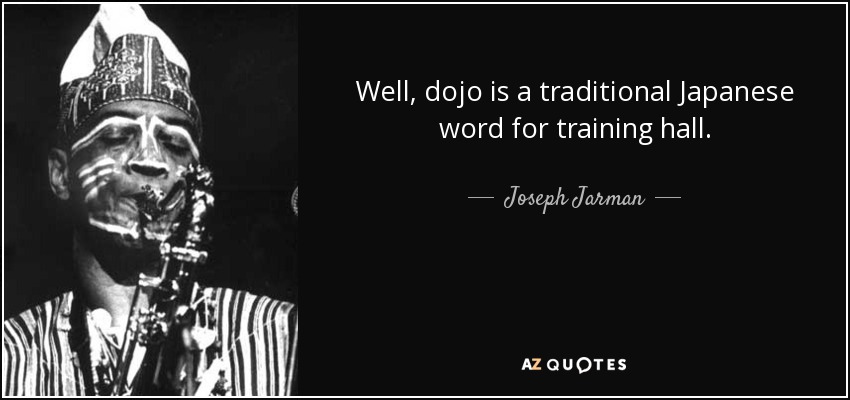This mini digital poster features a black background with a striking black-and-white composition. The left third of the poster showcases a black-and-white photograph of Joseph Jarman. Clad in a striped, possibly traditional, outfit and a decorative headdress, Jarman is seen playing a saxophone or a similar wind instrument. His face is adorned with horizontal stripes of white paint, adding a distinctive touch to his appearance. The right two-thirds of the poster are dedicated to a quote attributed to him, presented in white text: "Well, dojo is a traditional Japanese word for training hall." This quote is sourced from AZ Quotes, as indicated at the bottom of the poster. The overall layout emphasizes the bold contrast between the image and the text, lending a timeless and thought-provoking quality to the design.